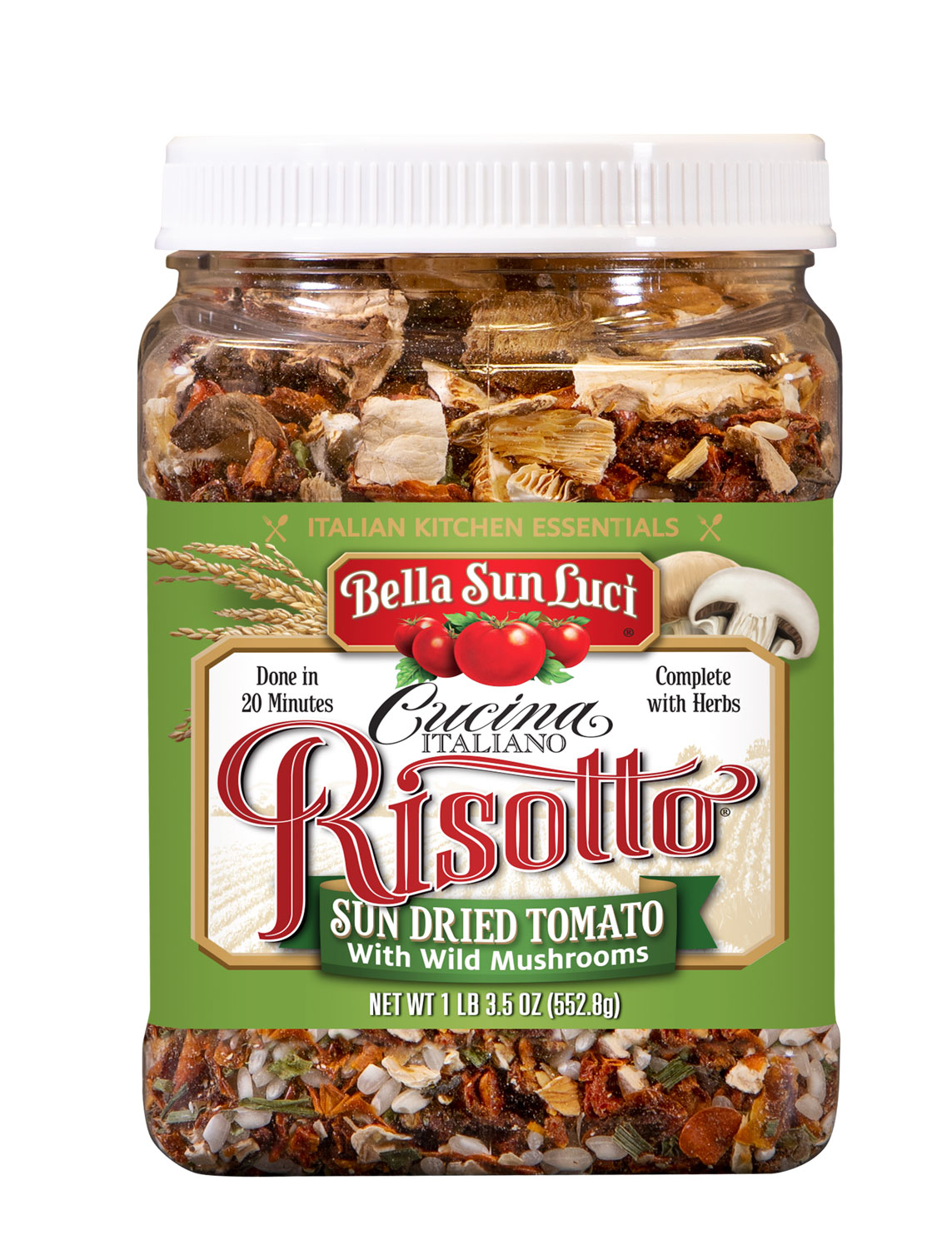The image features a square, clear jar with a white twist-on plastic lid. The jar contains a mix of various herbs, spices, rice, and sun-dried tomato pieces, prominently shown alongside large dried pieces of mushroom at the top. The label is a medium green with a red banner that has yellow text reading "Italian Kitchen Essentials." The red banner is outlined in gold and inscribed with "Bella Sun Luci" in white text. Images of tomatoes, mushrooms, and grains decorate the label, which also includes the text "Cucina Italiano Risotto," "Sun-Dried Tomato with Wild Mushrooms," "Done in 20 Minutes," and "Complete with Herbs." Additional details on the label list the net weight of 1 lb 3.5 oz (552.8 g). The overall aesthetic of the jar suggests a well-packaged culinary product, likely intended for making a flavorful Italian risotto. The background of the image is white, emphasizing the colorful and detailed design of the label and the contents of the jar.